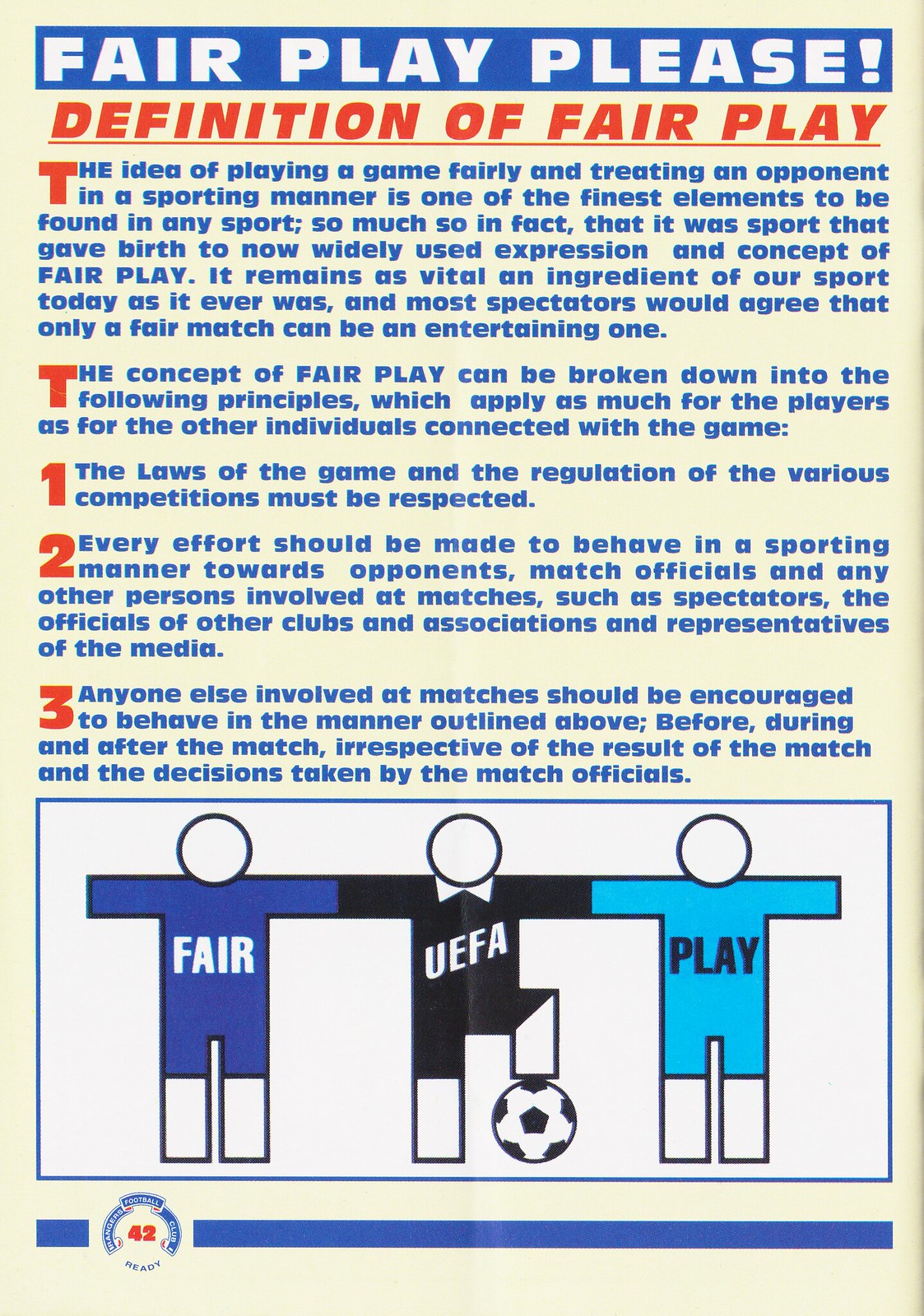This image is a promotional poster, likely from a football (soccer) program, designed to advocate for fair play. At the top, the poster features a blue rectangle with white text that reads "Fair Play Please." Below this title, the poster presents a detailed definition of fair play, articulated through an introductory passage and three key principles. The introduction emphasizes that playing a game fairly and treating opponents with respect is a crucial aspect of any sport, noting that fair play enriches the sporting experience for both participants and spectators. The principles outlined include respecting the game's laws and competition regulations, demonstrating sportsmanship towards all match participants and spectators, and encouraging such behavior consistently, regardless of the match outcome or officials' decisions.

Beneath the text, there is a diagram consisting of three caricatures—somewhat more detailed than stick figures but still simplistic, without facial features. These characters are standing arm-in-arm. The player on the left is wearing a blue jersey labeled "Fair," the player on the right is in a light blue jersey labeled "Play," and the central figure, dressed as a referee, has a jersey that reads "UEFA." The central figure has one foot up on a soccer ball. The poster prominently uses colors such as light blue, royal blue, red, and off-white.

Overall, this print clearly communicates the values and expectations of fair play within the sport, through both text and illustration, combining principles of sportsmanship with visual elements that highlight collaboration and fairness.